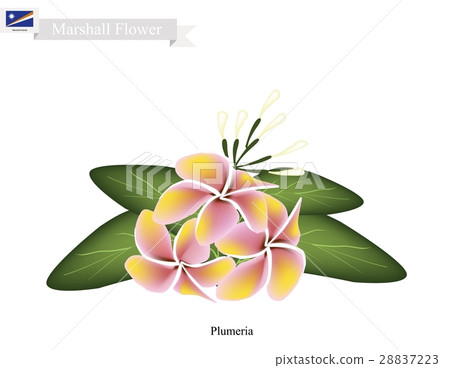This is a color drawing of a plumeria flower, depicted in a detailed, digitally created image commonly used as stock imagery. Dominating the center are four green leaves, with three pink flowers prominently displayed in front. Each flower boasts four to five light pink petals, accented by yellow centers. Some flowers also feature thin green lines with white tips extending from them. In the upper left-hand corner, a dark blue flag with a white circle, intersected by orange and white lines, is visible. This corner also features the text "Marshall Flower" in white lettering within a faint gray box. Below the central floral arrangement, the word “Plumeria” is written in small black letters. At the bottom, the watermark "pics2stock.com" followed by a numerical identifier is noted, indicating its stock photo origin. The predominant colors include blue, red, orange, yellow, gray, white, green, pink, and yellow. The overall aesthetic suggests it is a high-quality JPEG frequently hosted on image licensing platforms.